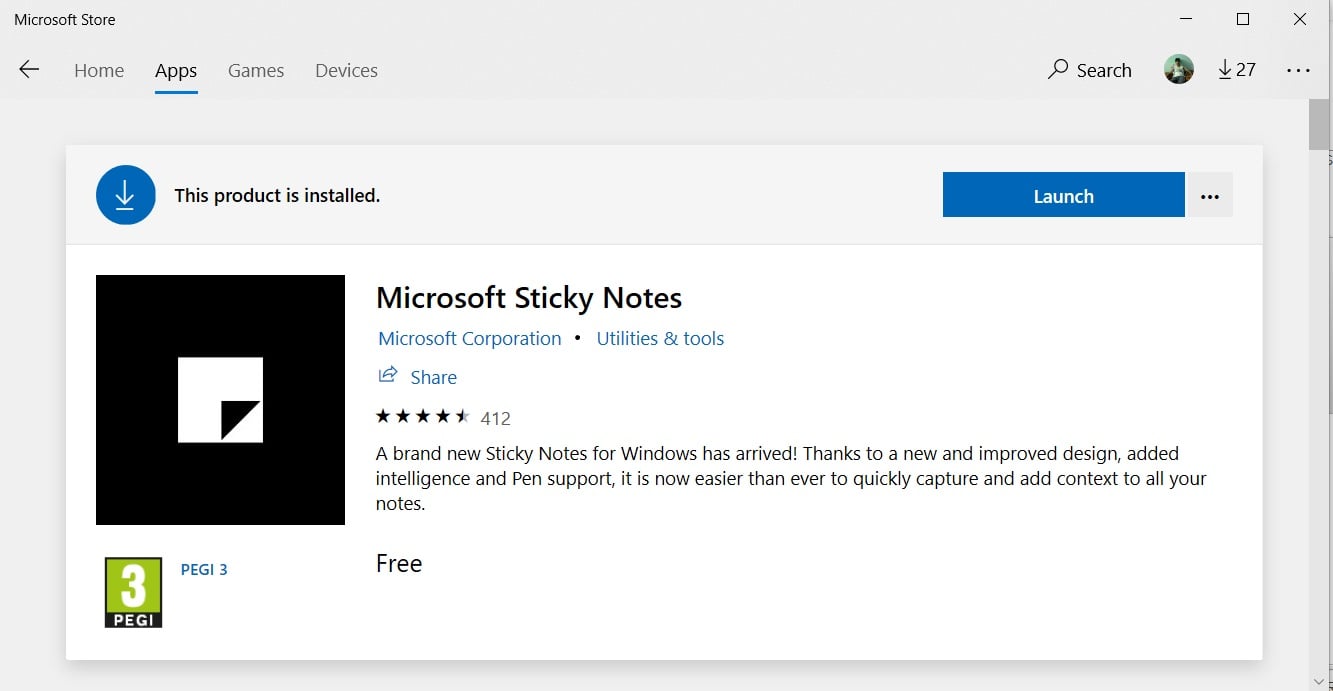The screenshot captures the Microsoft Store interface, where various UI elements are prominently displayed. At the top-left corner, the "Microsoft Store" label is clearly visible, signifying the application in use. On the top-right corner, three control buttons are aligned—an 'X' to close the window, a square for maximizing or minimizing, and a straight line for minimizing the window entirely. Just beneath these controls, an array of navigational elements is arranged: from left to right, an arrow for backward navigation, alongside tabs labeled "Home," "Apps," "Games," and "Devices." The "Apps" tab is highlighted with a darker shade and a blue underline, indicating the active page.

Further to the right on the same navigation bar, a search box is present, followed by a user avatar icon showing 27 downloads. Adjacent to the avatar, three dots suggest a dropdown menu for additional options. A scroll bar flanks the far right side of the window.

In the center of the page, detailed information about "Microsoft Sticky Notes" is displayed. This includes the app's publisher information, sharing options, user ratings, and pricing details. Notably, the product is shown as already installed on the user’s device, indicated by a message stating "Installed," accompanied by a prominent blue "Launch" button.